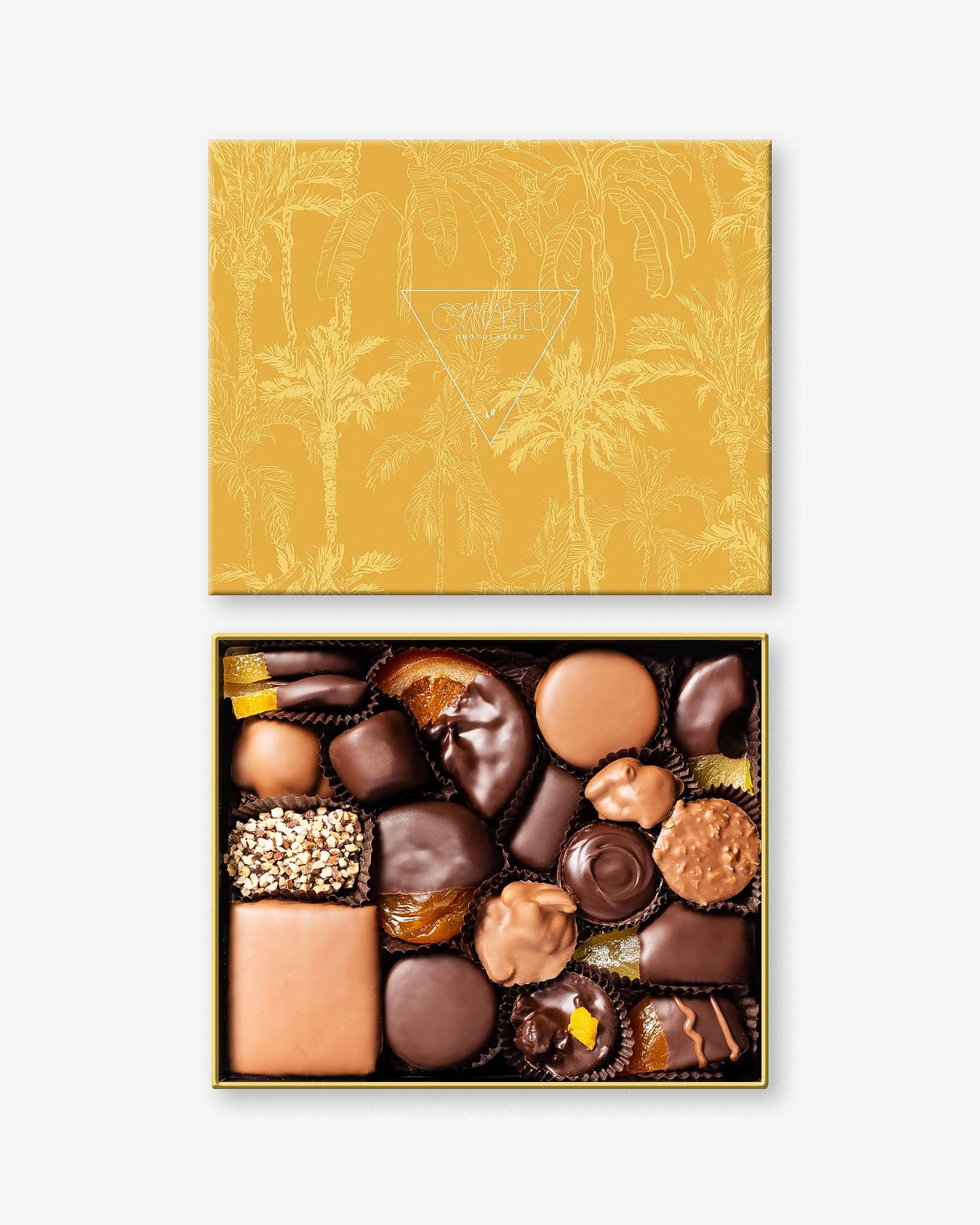This image depicts a meticulously curated box of chocolates and treats arranged on a light gray or off-white surface, either a table or countertop, photographed indoors. The scene is vertically aligned, showing the open box with the lid positioned above it. The lid is predominantly gold with a pattern of light gold palm trees and features a central, downward-pointing white triangle with faint, unreadable writing inside. The rectangular box, bordered in gold, houses roughly 20 assorted chocolates and candy-like treats, each nestled in a dark brown cup. 

The lower left of the box contains a large light brown square of milk chocolate, while the upper right holds a similarly sized light brown circle. To the left of this circle, there is a slice of orange, partially dipped in chocolate with its sugared segment exposed. Additional pieces include fruit slices like papaya or pineapple with parts left uncoated, scattered light to dark chocolate varieties, caramel confections, and nut-studded chocolates, including a peanut butter cup on the far right. The detailed assembly and diverse selection highlight the visual appeal and luxurious nature of this chocolate box.